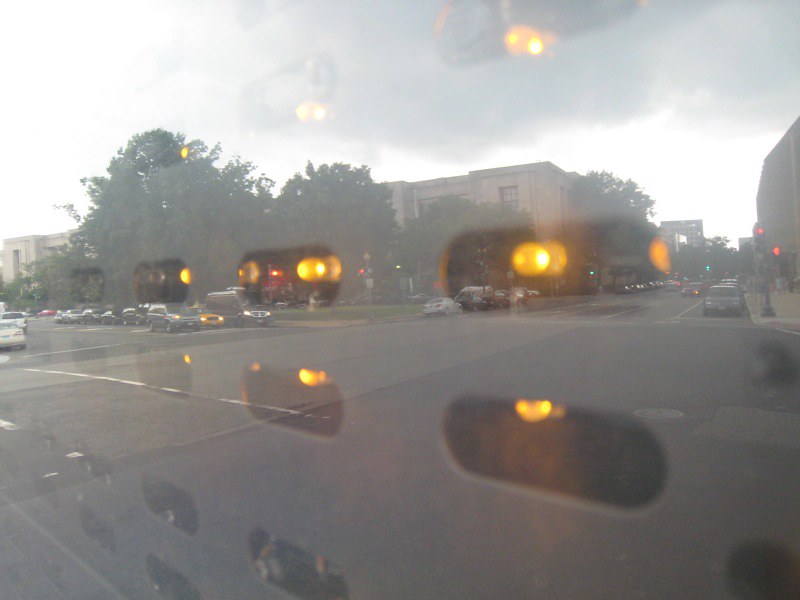The photograph captures a scene viewed through a vehicle or house window, evidenced by the visible glare showing oblong shapes with lights in their centers. Outside the window, a bustling intersection unfolds where two streets meet at a right angle. The street in the foreground extends to the left, while another street branches off to the right. There's a notable amount of traffic, with numerous cars parked along the sidewalks.

In the background, a patch of grass and several trees provide a touch of nature amidst the urban setting. Beyond this, beige buildings are visible, evoking the appearance of a college campus. The sun's light creates reflections on the window, adding a layer of depth to the image. The scene is vibrant with the everyday life of what appears to be a busy urban or campus area, combining the elements of nature, architecture, and human activity seamlessly.